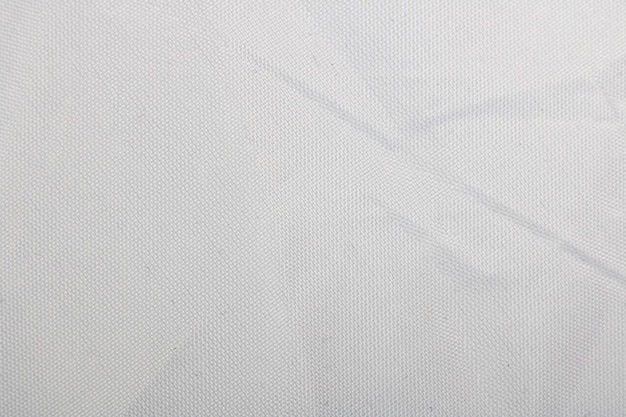The image showcases a close-up view of a piece of white fabric or cloth, exhibiting a subtle texture reminiscent of woven threads. Its surface features a gradient from very light grey at the top to a slightly darker grey at the bottom. Numerous creases accentuate the fabric’s texture, with some notable wrinkles concentrated near the right edge. One prominent crease extends almost diagonally from the bottom right to the middle of the upper section, flanked by more subtle creases on either side. The overall appearance is that of a softly nubby, textured material with visible wrinkles that lend a sense of depth and dimension. The entire scene is set against a nearly white background, creating a minimalistic yet detailed composition.